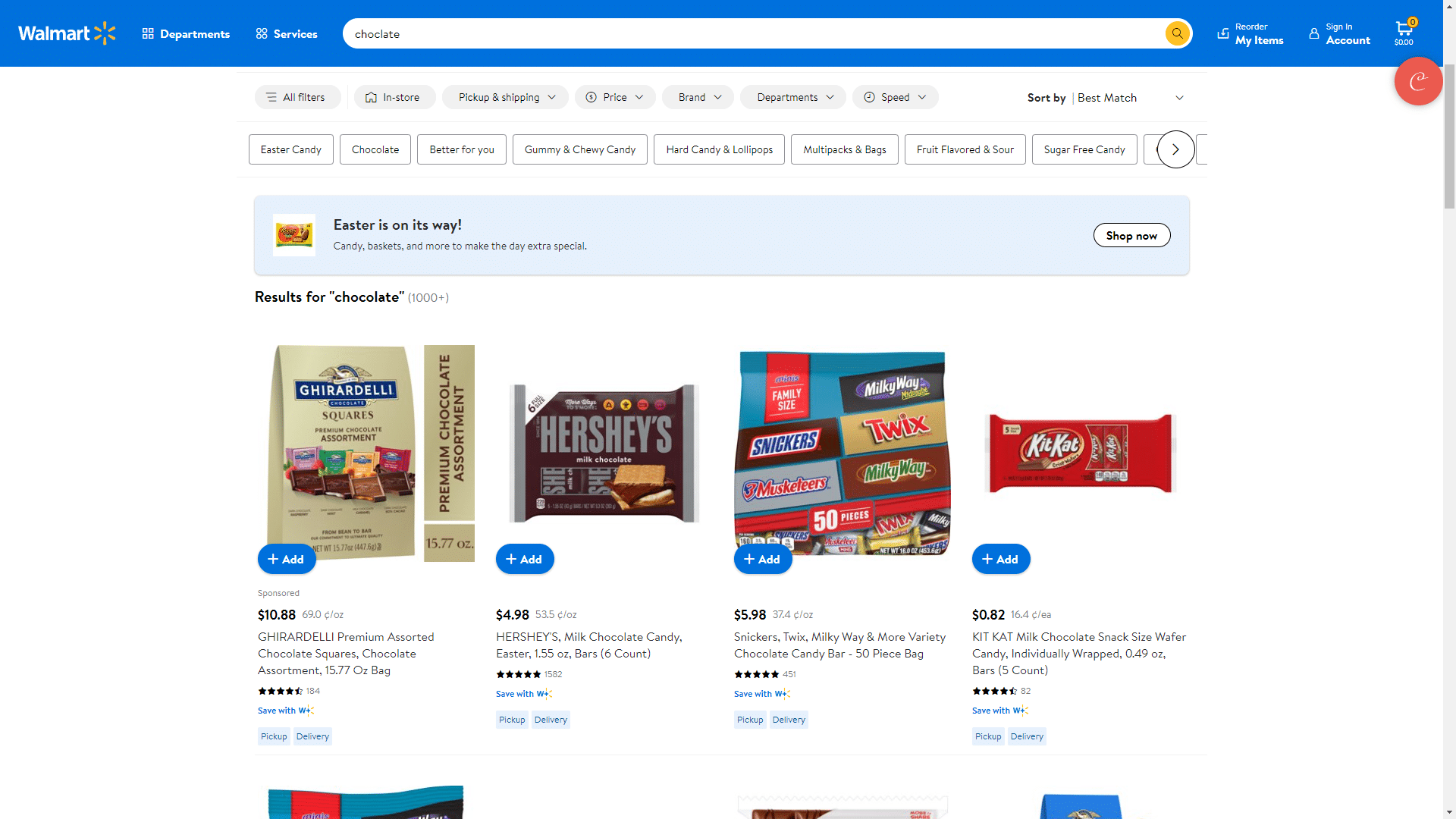The image depicts a webpage with a white background. At the top of the page, there's a bold bright blue banner featuring the Walmart logo in white text. Adjacent to the logo is the recognizable yellow sunburst icon. Below the banner, the site showcases 11 department categories, followed by text too small to discern. A search box occupies the center space with a yellow circular magnifying glass icon at its right end. To the right, "My Home" is displayed, and beside it is a miniature shopping cart icon highlighted with a small yellow circle. Next to this, there's a red circle containing the letter "E."

Further down on the webpage, across the white background, there are several navigational headings. A "Sort By" field with a selection box is present along with additional administrative headings and a circular icon featuring a right arrow, enabling more navigation options.

Midway through the page, a prominent blue box is visible containing a smaller yellow box with the text "Easter is on its way" along with a white "Shop Now" button.

Below this, the white background displays search results for "Chocolate." The first product listed is Ghirardelli chocolates, with a blue "Add" button. Following are Hershey's chocolates, a variety pack including Snickers, Three Musketeers, Twix, and Milky Ways, each accompanied by blue "Add" buttons. Similarly, Kit Kats are displayed with a corresponding blue "Add" button. The top portion of three additional products is partially visible. Towards the right side of the page, there's a gray vertical slider for navigation.